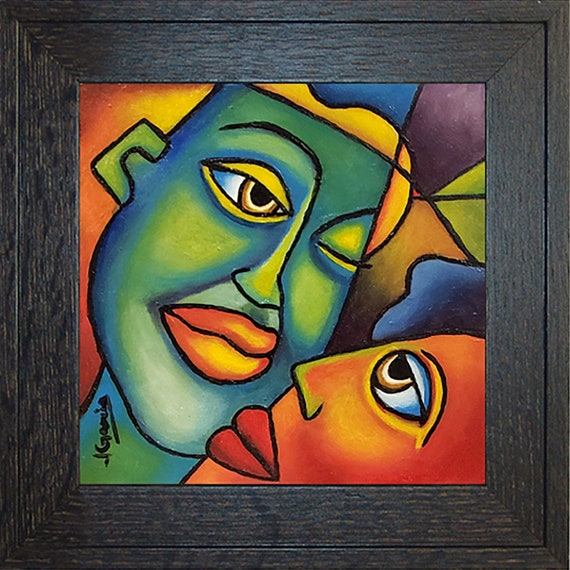This is a detailed depiction of a framed cubist painting centered within a polished, dual-layer wooden frame that appears black or dark grey, preserving some of the wood's natural details. The painting itself is square and predominantly features two abstract, geometric portraits reminiscent of Picasso's style. The face on the left is painted predominantly in blue and green shades with some yellow, while the face on the right predominantly uses orange and red hues. Geometric patterns and vibrant colors fill the background, interspersed with black lines. The facial expressions suggest that the two faces are staring at each other. Positioned slanting to the right, the first face occupies the middle-right of the painting, while the second face is at the bottom-center, slanting towards the right corner. There is an indistinguishable signature on the bottom left, beginning with what appears to be a letter "G."